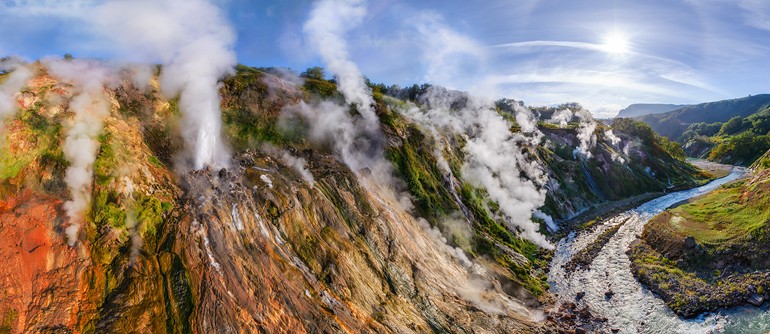In front of us is a picturesque and colorful photograph of tall, rocky mountains viewed from a high vantage point, giving us an almost aerial perspective. The scene is set in daylight, with a bright blue sky accented by faint white clouds and the sun positioned towards the right. The mountains feature a dramatic display of colors and textures: the near cliff sides are brown and coral-colored, with patches showing eroded reddish hues and scattered green vegetation. White smoke or steam is visible drifting from the mountainside, adding a surreal touch to the landscape. Descending from the rocky heights, the mountains give way to a winding river at the bottom, its waters briskly moving and churning white foam over the visible rocks. To the right of the river, the land transitions to green, grassy knolls, indicative of a summer setting. In the distance, a series of hills and mountains provide a majestic backdrop to this serene and vibrant natural scene.